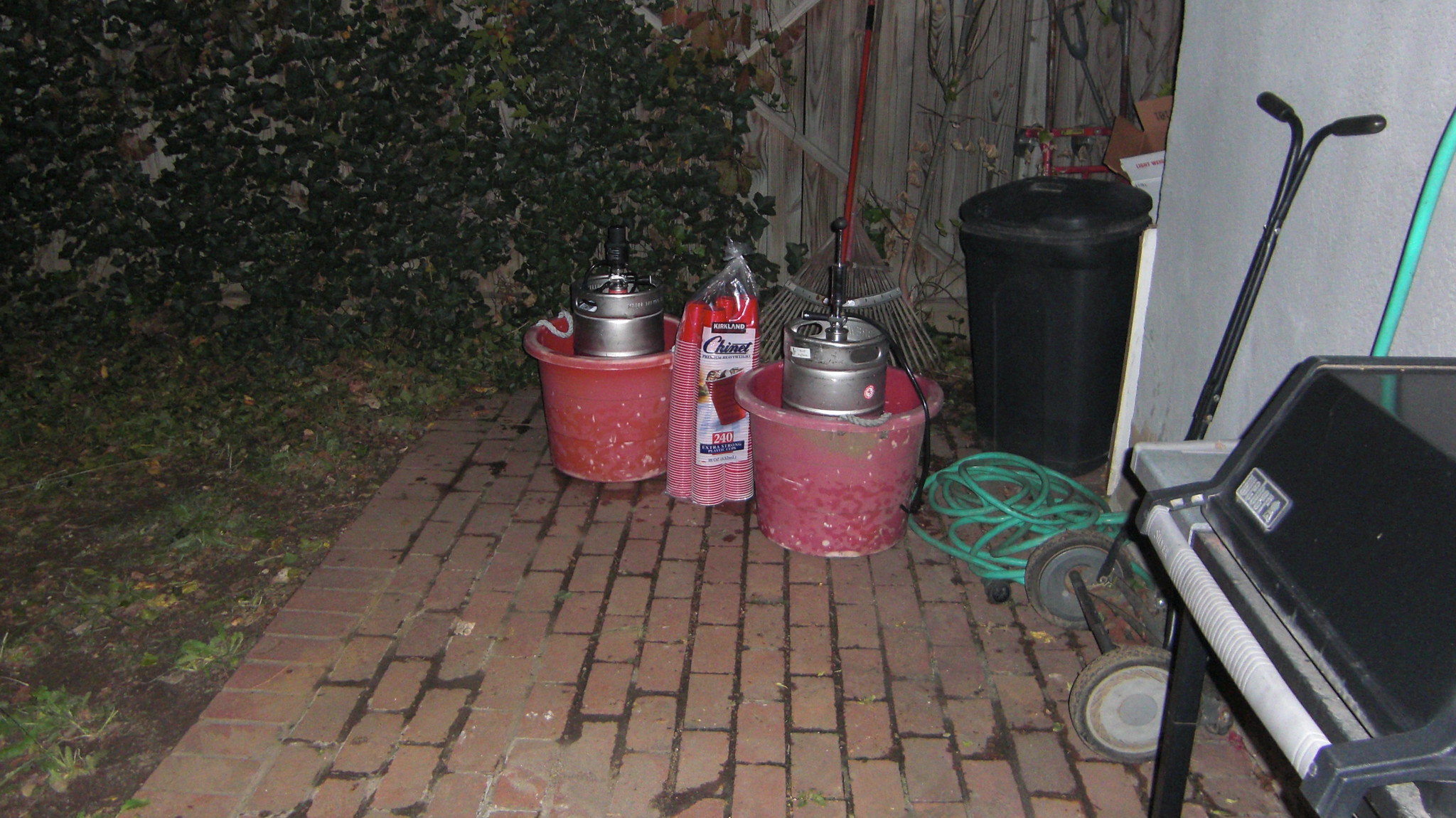This is a detailed nighttime color photograph of a backyard patio area. Dominating the center of the image is a red brick path, flanked on the left by a patch of green grass and dirt, leading up to a wooden fence. The fence on the top left corner is partially covered in green leafy vines. On the patio, there are two large, dirty red buckets, each holding a metal beer keg. Between these buckets is a packet of Kirkland brand red plastic cups, prominently displaying "C-H-I-N-E-T" and advertising 240 extra strong plastic cups with an image of an ice-filled cup on the front label. To the right of the kegs is a coiled green garden hose and a tall black plastic trash can. Further to the right, against a white building wall, there's a push mower and a Weber grill. In the back, a rake with a red handle is leaning against the wooden fence. The entire scene is framed in a rectangular shape.